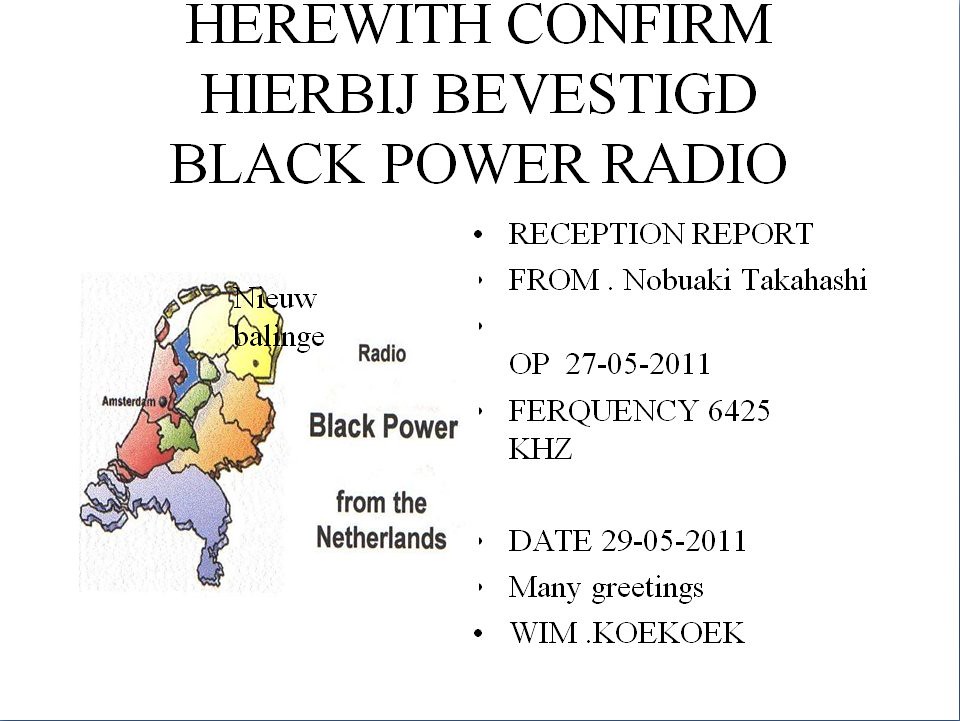The image displays a scanned card sent to a shortwave radio listener, featuring text and a colorful map. At the top, it reads "Herewith Confirm" alongside the Dutch words "Hierbij Bevestigd," indicating confirmation. Below this, the card identifies itself as a reception report from Nobuaki Takahashi, dated May 27, 2011, with the frequency listed as 6425 kHz.

On the left side, there's a vibrant map comprising several connected countries in varying shades of purple, orange, red, green, blue, and yellow, each separated by lines. The card's design is predominantly white with black text, and it prominently mentions "Radio Black Power from the Netherlands." At the bottom, it includes greetings from Kim Koke, dated May 29, 2011. This card acts as a thank you note, confirming that the listener's report has been acknowledged.